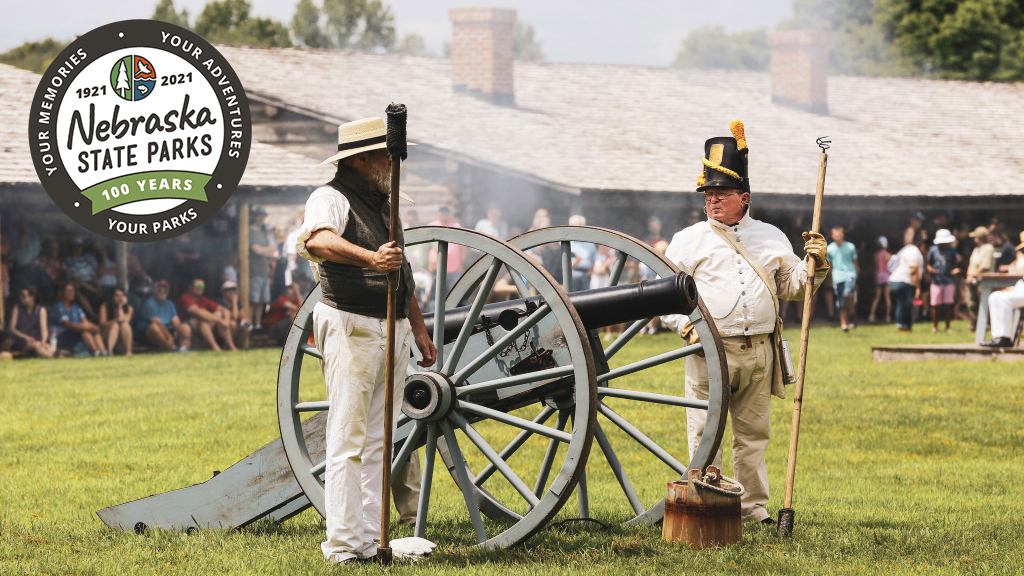The photograph captures an outdoor scene at a historical reenactment event, likely part of a celebration for Nebraska State Parks' 100th anniversary (1921-2021). Central to the image are two men positioned on either side of a cannon with large wheels, each holding tools used to handle gunpowder and clean the cannon's muzzle. Both men are wearing hats; their attire is not distinctly from any particular historical period, yet they seem to be demonstrating the firing process. The scene includes well-manicured grass, a wooden bucket in front of the cannon, and a sizable structure with a large roof and porch in the background, offering shade to seated spectators. In the upper-left corner, a circular emblem displays the text in white letters on a black border, "Your Memories, Your Adventure, Your Parks." Inside the circle, against a white background, are the dates "1921" and "2021," alongside a small circle featuring a tree, bird, and fish icon, signifying the Nebraska State Parks' centennial commemoration. Below the circle, a green banner reads "100 years." The atmosphere is sunny, highlighting the celebratory and educational essence of the event.